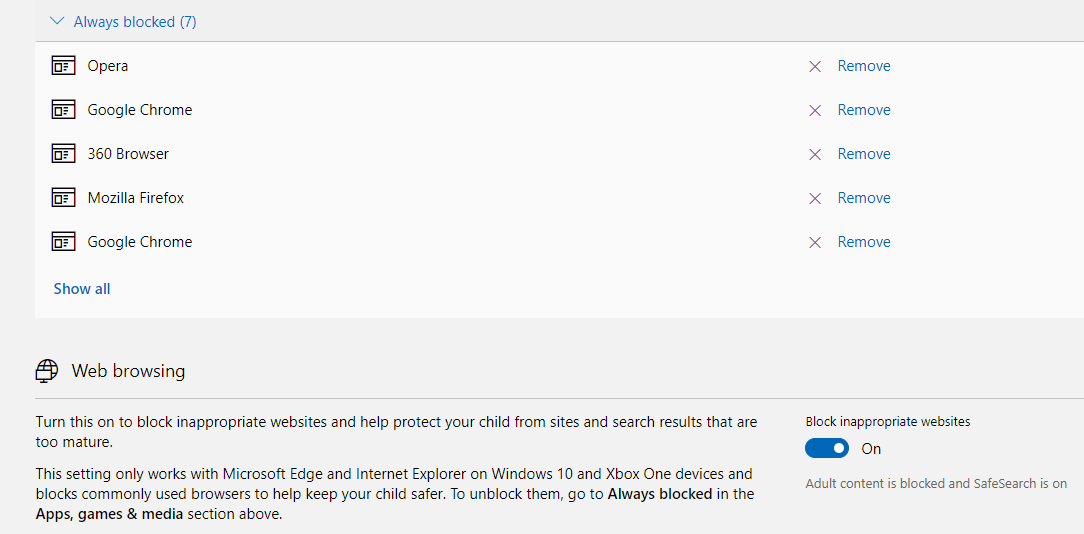This image is a horizontal screenshot of a webpage dedicated to blocking websites, featuring a primarily white background accented by a thin grey banner at the top. Within this banner is the text "Always blocked" accompanied by a down scroll button and the number (7) in parentheses, indicating the number of blocked sites.

In the main section of the page, a list of blocked browsers is prominently displayed, including Opera, Google Chrome (appearing twice), 360 Browser, and Mozilla Firefox. Each entry has a corresponding small "X" and "Remove" option located in the right-hand column, allowing users to manage the list of blocked websites.

At the bottom of the image, on a very light grey background, there's an informative section titled "Web browsing." This section advises users that they can turn on the feature to block inappropriate websites, thereby protecting children from mature content. It specifies that this setting is effective only with Microsoft Edge and Internet Explorer on Windows 10 and Xbox One devices, and notes that commonly used browsers are blocked to enhance child safety. To unblock any of the listed websites, users are directed to the "Always blocked" section within the apps, games, and media settings above.

In the lower right-hand corner of the screen, there is a blue slider button labeled "Block inappropriate websites," which is currently set to "On." Below this, further clarification states that adult content is blocked and safe search is activated.